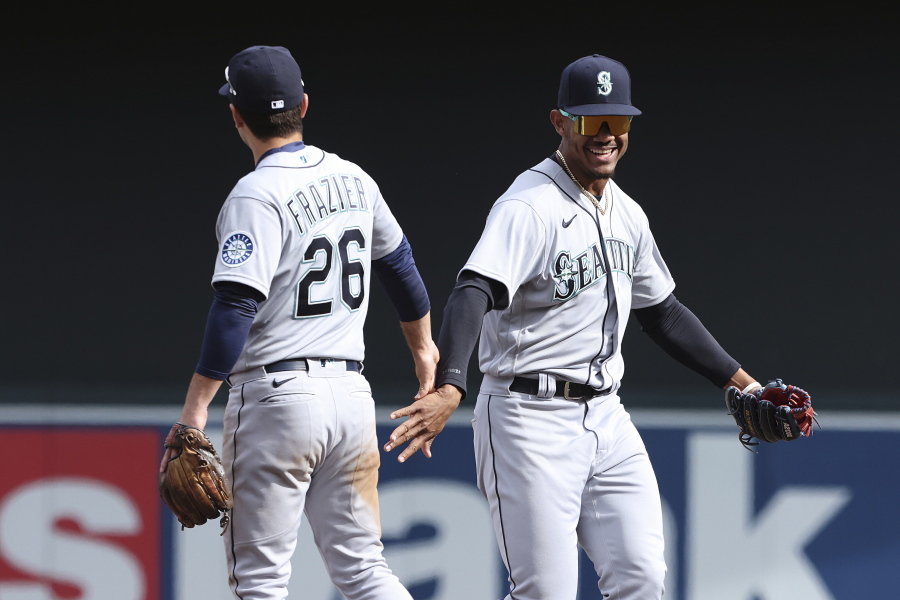This detailed sports photography captures a moment between two Major League Baseball players from the Seattle Mariners, both wearing their team's gray Nike uniforms. The player on the left has his back to the camera, revealing his name, "Frazier," and the number 26 on his jersey. He dons a navy Seattle hat and gray pants, completing his attire with a brown leather glove. To his right, a teammate faces the camera, identifiable by his reflective, heavy-shaded sunglasses and navy Seattle hat. He also wears a matching gray uniform and grips a blue and red glove, possibly holding a baseball. The players appear to be celebrating a successful play, exchanging a waist-level high-five without making eye contact. The background is largely nondescript, featuring some advertisements and a wall, placing the focus squarely on the athletes' camaraderie and their on-field moment of triumph.